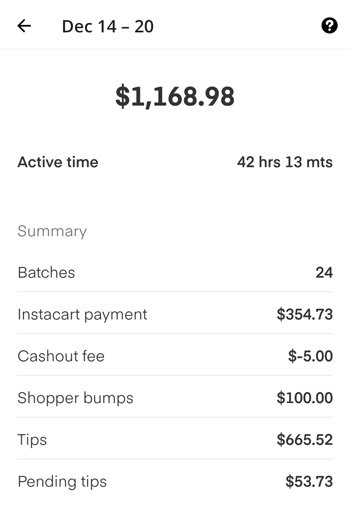**Caption:**

The screen displays the earnings summary for an Instacart shopper from December 14th to December 20th. Key elements of the interface include a back arrow and a black circle with a white question mark, indicating help or additional information is available.

The earnings breakdown is as follows:
- **Total Earnings:** $1,160.90
- **Active Time:** 42 hours and 13 minutes
- **Number of Batches:** 24
- **Instacart Payment:** $354.73
- **Cash Out Fee:** -$5.00
- **Shopping Bumps:** $100.00
- **Tips:** $665.52
- **Pending Tips:** $53.73

The figures are clearly displayed in black text against a white background, making them easy to read. The layout effectively shows the total amount earned and provides a comprehensive breakdown of earnings, including base payments, tips, and additional fees. To seek help or ask questions, users can click on the white question mark in the black circle.